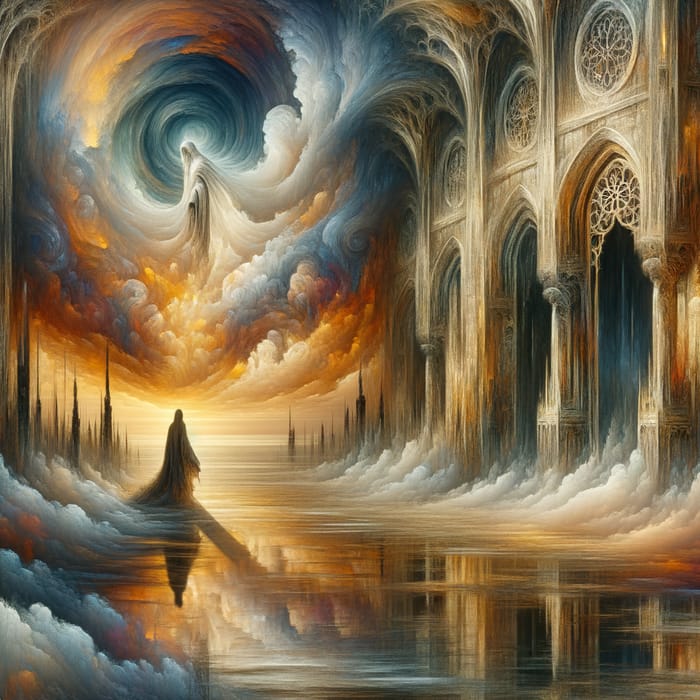This fantasy-style painting, created with what appears to be acrylics, features a mesmerizing gothic cathedral situated in the top right portion. The cathedral's front wall is adorned with grand pillars, each crowned with intricate stonework that seamlessly transitions into the form of melted trees. These trees spiral upward, merging into a swirl of blue and white clouds, which then transform into a vortex of blue and orange hues. At the heart of the vortex is a draped, ethereal figure, evocative of the Virgin Mary, adding a sacred and tranquil presence to the scene.

The base of the cathedral wall is enveloped in clouds that transition into puddles, creating a reflective surface reminiscent of melted ice or rain. Spires dart into the distance on both the left and right sides, further enhancing the sense of depth and gothic grandeur. On the left side of the painting, another draped figure, dressed in a long gown and carrying religious overtones, stands gracefully. This figure's image, along with the cathedral and the surreal clouds, is beautifully mirrored in the reflective, watery ground, giving the entire composition a dreamlike and mystical ambiance.